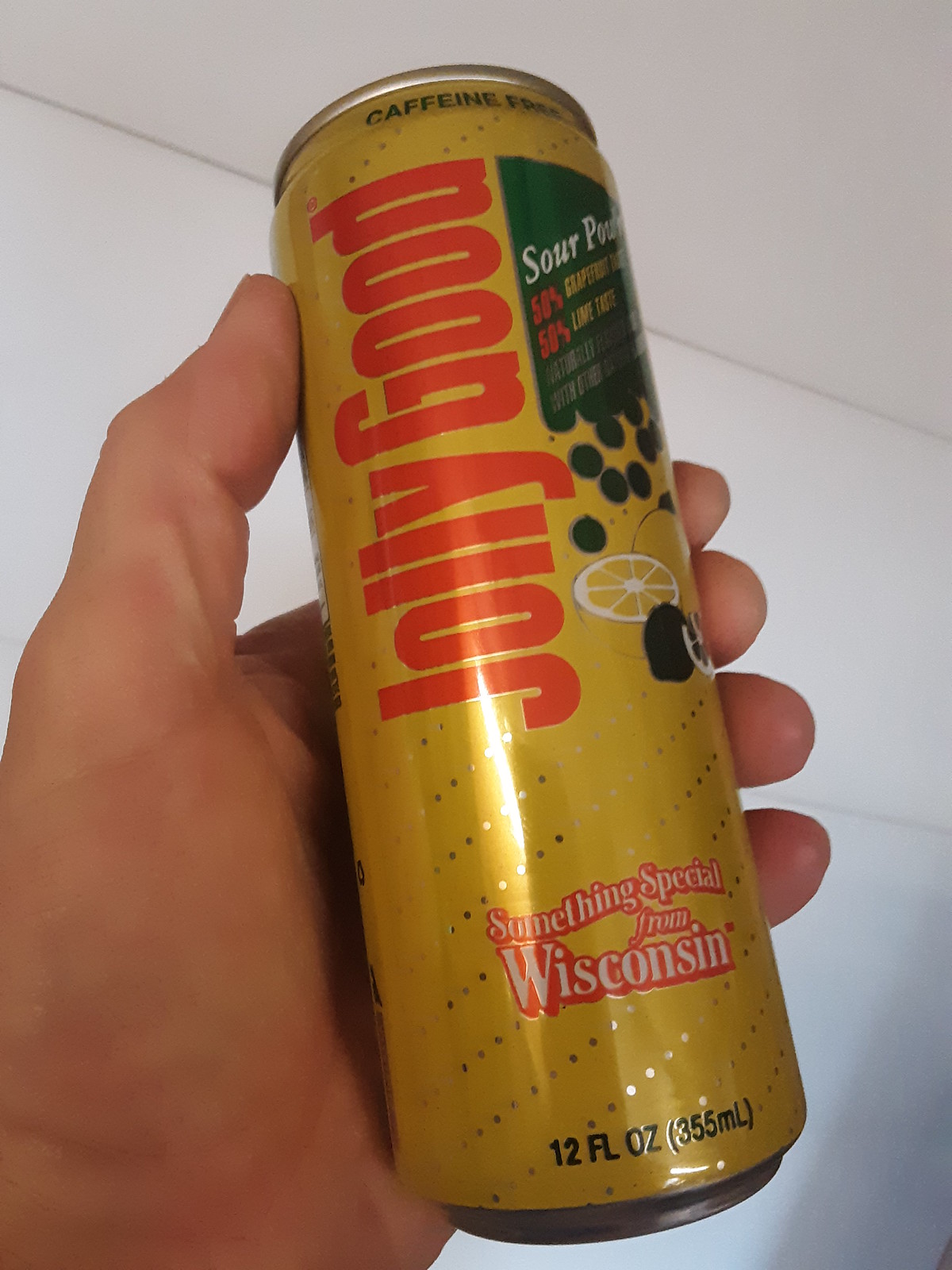This photograph captures a close-up of a man's hand, likely Caucasian, with short fingernails, holding a beverage can. The background is a stark, clean white, suggesting a white wall and ceiling. The can, distinctly highlighted against the plain backdrop, holds 12 fluid ounces of a beverage. It features a dark yellow color adorned with gold dots arranged in diagonal stripes.

The brand name, "Jolly Good," is prominently displayed in large, red letters running vertically along the can's side, making it readable if the can were laid on its side. Adjacent to the word "Good," there is a solid green rectangle containing the words "Sour Punch" in white font with a red outline. From the letter "D" in "Good" extending downward to the "G," the green transitions into green circles merging with the can’s main yellow color, incorporating images of a lemon and lime slice.

At the bottom of the can, the words "Something Special from Wisconsin" are also noted in white letters with a red outline, adding a regional touch to the product's description.